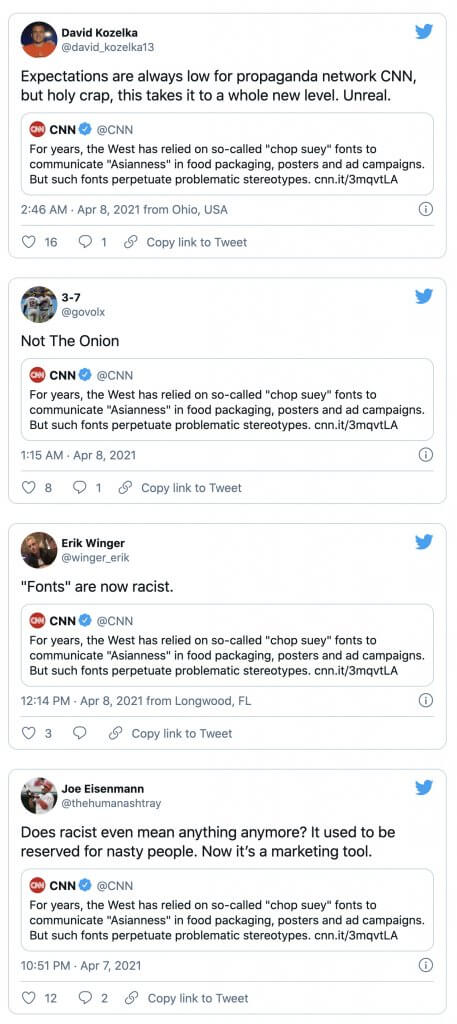This image portrays a series of four Twitter messages displayed on a clean, white background. Each tweet originates from a different individual, identifiable by their respective photo icons positioned at the top left of their messages, their names adjacent, and their Twitter handles beneath. The distinctive blue bird icon of Twitter appears on the top right corner of each tweet.

The topmost message is from David Kozileka (@david_kozileka3) and reads: "Expectations are always low for propaganda network CNN, but holy crap, this takes it to a whole new level, unreal." Embedded within his tweet is the original CNN message: "CNN, for years, the West has relied on so-called chop suey fonts to communicate the Asian-ness in food packaging posters and ad campaigns, but such fonts perpetuate problematic stereotypes. CNN.it/3MQVTLA." This tweet was posted at 2:46 a.m. on April 8th, 2021 from Ohio, USA, and includes indicators for the number of likes, comments, and an option to copy the tweet link.

The second message comes from @3.7_NOT_THE_ORION, who retweeted and quoted the same CNN message, posting their response at 1:15 a.m. on April 8th, 2021.

The third tweet is authored by Eric Winger (@ericwinger), and reads: "Fonts are now racist," also referencing the CNN message mentioned above. This was posted at 12:14 p.m. on April 8th, 2021 from Longwood, Florida.

The final message is from Joe Eisenman (@joe_eisenman) and states: "Does racist even mean anything anymore? It used to be reserved for nasty people. Now it's a marketing tool," once again quoting the CNN message. Joe’s tweet was posted at 10:51 p.m. on April 7th, 2021, and, similar to the first tweet, it includes indicators for how many people liked and commented.

Each tweet displays the typical Twitter functionalities such as the number of likes, comments, and an option to copy the tweet link, providing a snapshot of the ongoing conversation reacting to the CNN post about culturally sensitive font usage.